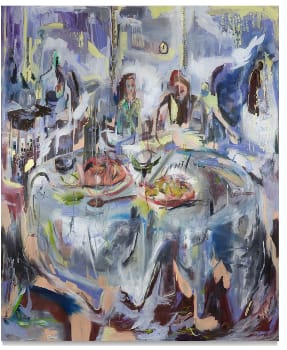This is a highly stylized, abstract painting reminiscent of the works of Salvador Dali or Picasso, capturing a surreal dining scene. The focal point is a large, round table viewed from the front, adorned with various foods, drinks, and a tablecloth. Seated at the table are two women, one on the left wearing turquoise with brown hair and appearing smaller, and another on the right dressed in white with gingerish-brown hair. The entire scene is enveloped in a dream-like, melted effect, with blurred, warped, and blended details, creating an otherworldly atmosphere. The background features dusky, shaded hues of purple, yellow, white, and dark blue, contributing to the painting's overall abstract and surreal nature. The dominant blue tones may evoke a sense of melancholy, reminiscent of pieces from Van Gogh's or Picasso's blue periods.